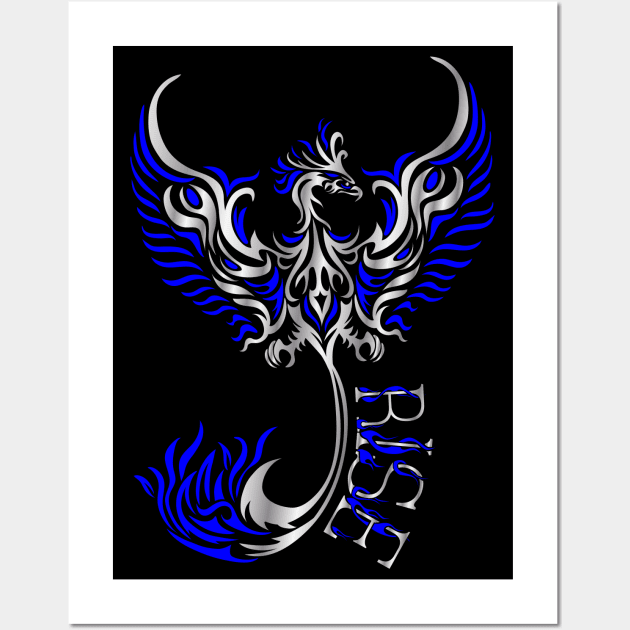This is a detailed and vibrant illustration mounted on a grey wall and encased in a white frame. At its center, the illustration features a majestic phoenix depicted in hues of metallic silver and a vibrant blue. The phoenix, with its head held high and facing to the right, spreads its intricately patterned wings symmetrically across the canvas. Each feather of the bird is meticulously designed, presenting an almost 3D appearance with lighter to darker grey transitions. The long, elaborate tail of the phoenix cascades downward, intertwining with blue flames, adding to the mythical and rebirth symbolism of the creature. The bird's claws are clearly visible, anchoring it in the midst of this dynamic display. At the bottom center of the image, the word "RISE" is artistically inscribed in metallic silver letters, encircled by blue lines that mimic the arc of the phoenix's tail, reinforcing the theme of resurgence. The entire scene is set against a striking black background, enhancing the clarity and brilliance of the illustration, and is well-lit to highlight the intricate details and vibrant colors.